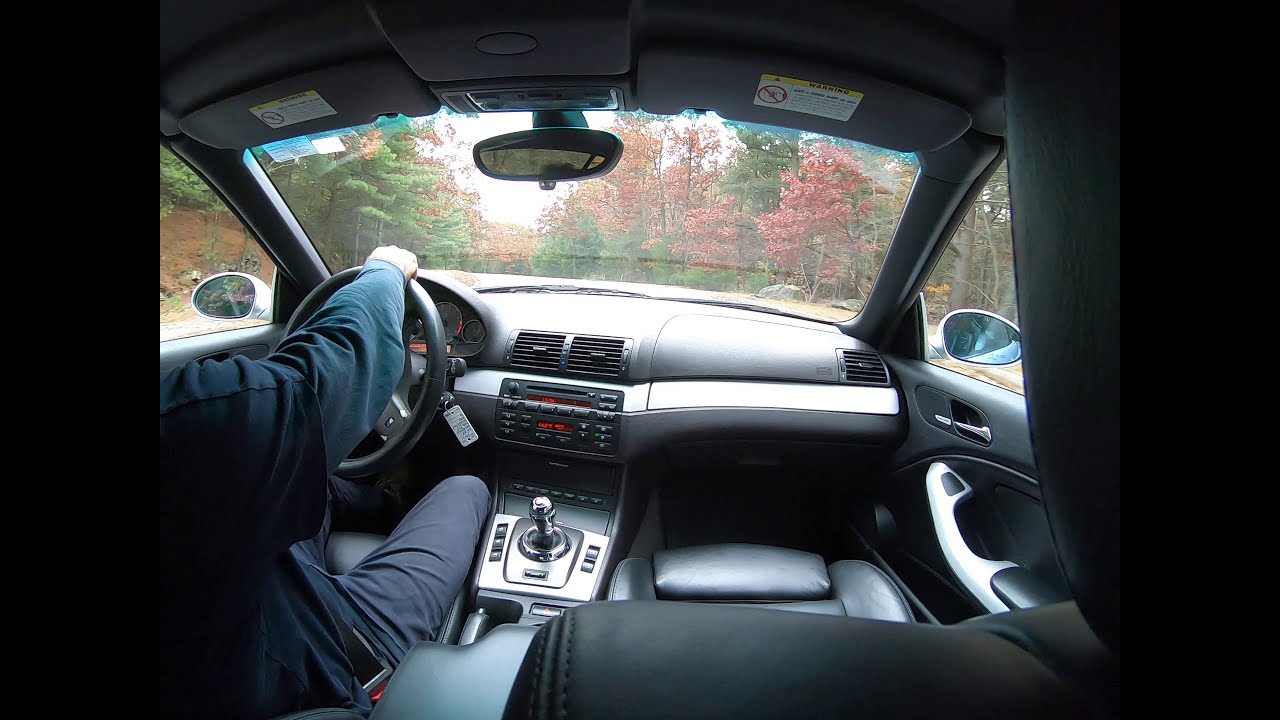This photograph captures the interior of a car traveling down a road bordered by tall trees, which display a vivid mix of green, red, and orange leaves. Taken from the back seat on the passenger side, the image provides a detailed view of the car's interior and its occupants. On the left, a Caucasian driver is visible, wearing black pants and a layered black outfit consisting of a short-sleeved T-shirt over a long-sleeved shirt. Their hand rests on top of the steering wheel. The photograph includes the front half of the car, showcasing the AC and radio system, gear shift, and an empty, black leather passenger seat. The dashboard and the outside scenery are visible through the front and side windows, providing a sense of motion and the vibrant autumnal landscape. The picture is framed with black vertical borders on either side, adding to the compositional structure of the image.